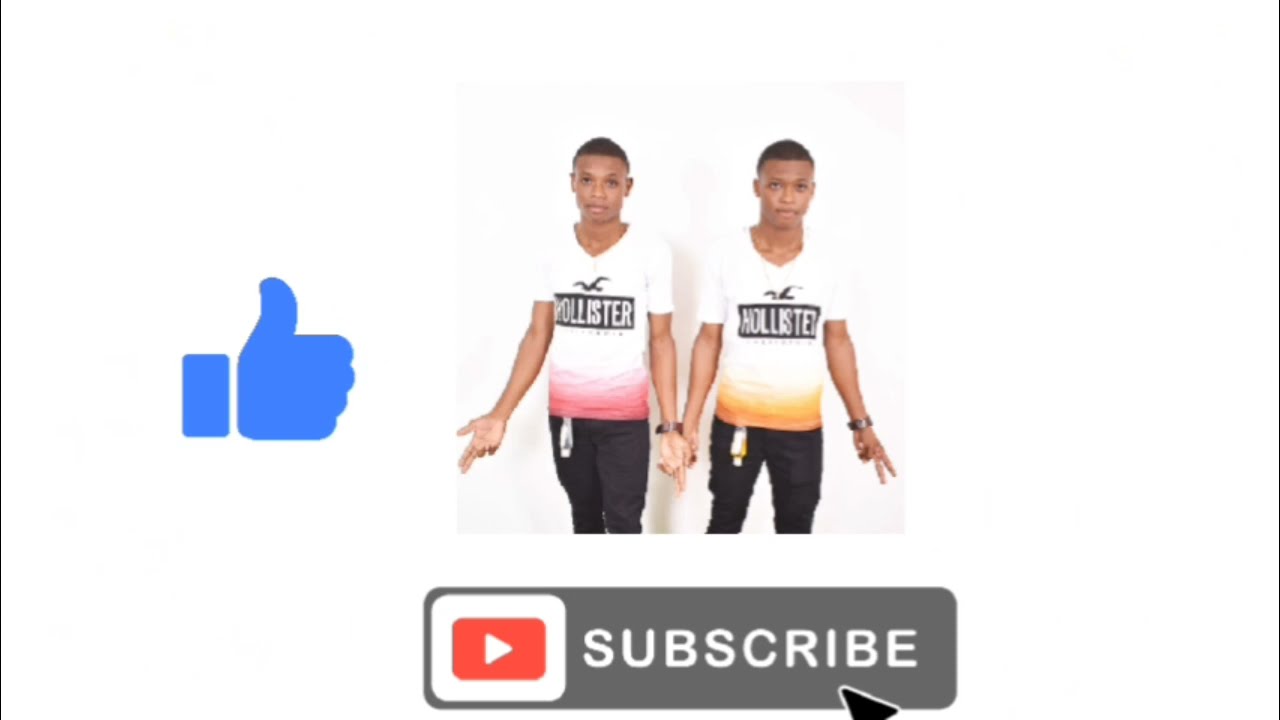The image features two young African American men standing side by side against a minimalist off-white background, enclosed by thin black borders on the far left and right sides. Each man dons a short-sleeved white Hollister t-shirt, emblazoned with a black rectangular strip displaying the brand's name in white text and a bird logo above. The man on the left sports a t-shirt with a pinkish-red band along the bottom hem, while the man on the right has a similar shirt but with an orange-yellow band. Both men wear black pants and have short black hair, enhancing their striking resemblance, suggesting they might be twins. They stand with their hands closest to each other overlapping, and their other arms outstretched with palms facing inward for the man on the left and downward for the man on the right. Beneath their feet, a gray rectangular box showcases the word "subscribe" in white letters, next to the YouTube logo—a red rectangle with a white play triangle in the center. On the left side of the image, midway up the frame, there is a prominent blue thumbs-up symbol, adding a social media element to the scene. This array of elements suggests that the image could be a promotional shot, possibly aimed at enhancing a YouTube channel.